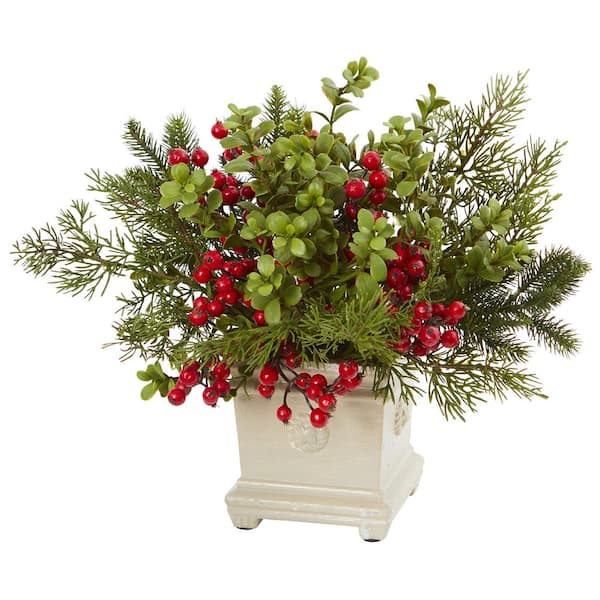In this image, we see a decorative indoor plant arrangement in a white, cube-shaped planter that features ornate texturing and emblems on its sides and stands on four small feet with dark felt at the bottom. The arrangement consists of a mix of foliage, including fir tree-like evergreen branches, rounded green leaves, and sprigs adorned with red berries. The combination of elements and their plastic-like appearance suggests that it might be an artificial plant, designed to resemble a holiday-themed decoration that doesn't correspond to any single real-world plant. The overall effect is a striking arrangement of green and red hues contrasted against a white background, creating a festive and visually appealing display.